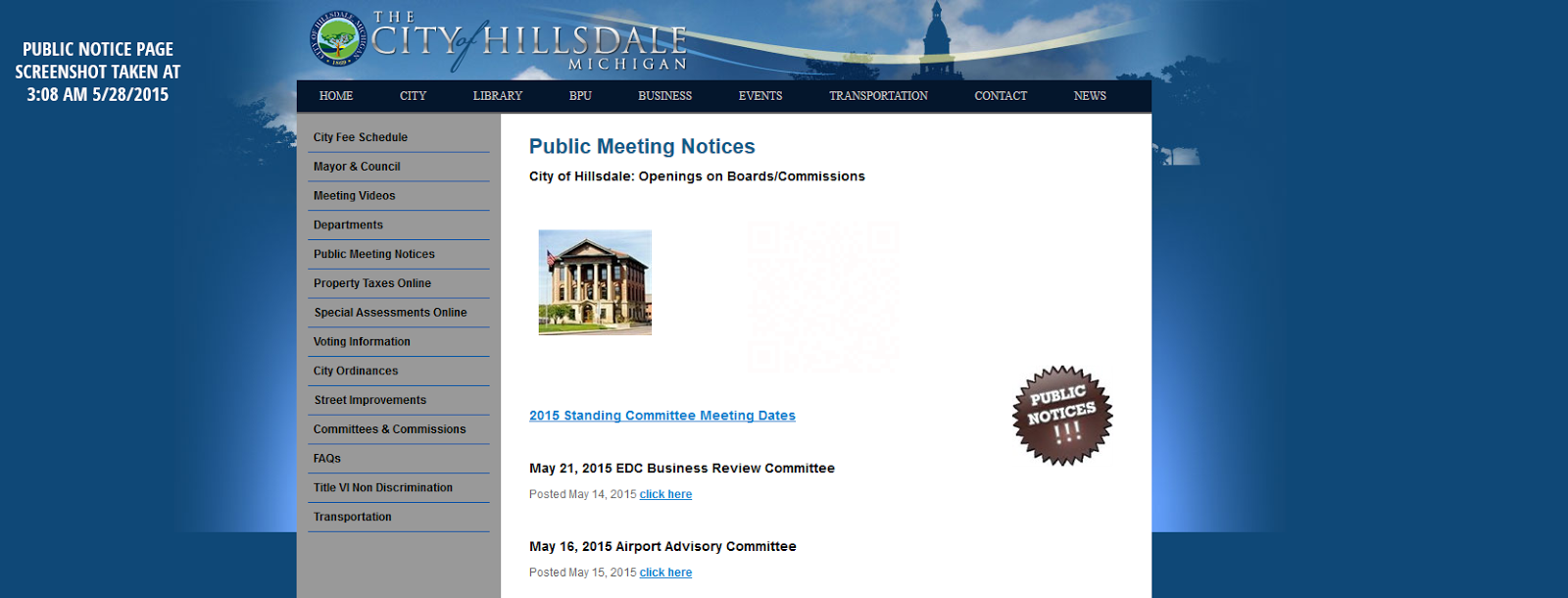This screenshot captures the official website of the City of Hillsdale, Michigan. The webpage features a blue background, and prominently displayed in the center is a box containing key information. The top left corner of the page includes a white section for public notices. The screenshot was taken at 3:03 a.m. on May 28, 2015. The title at the top reads "The City of Hillsdale, Michigan," accompanied by the city's official seal.

Beneath the title is a chart with a black header, which acts as a navigation menu. This header comprises approximately six tabs labeled: Home, City, Library, Events, Transportation, Contact, and News. The chart itself is divided into two panels. The left panel is gray and lists more than ten items, while the right panel features a white background. 

The right panel is titled "Public Meetings Notices: City of Hillsdale Openings on Boards and Commissions." Below this title, there is an image of what appears to be the City Hall. Underneath the photo, there is a hyperlink that reads "2015 Convenience Meeting Dates," which lists the dates May 21, 2015, and May 19, 2016.